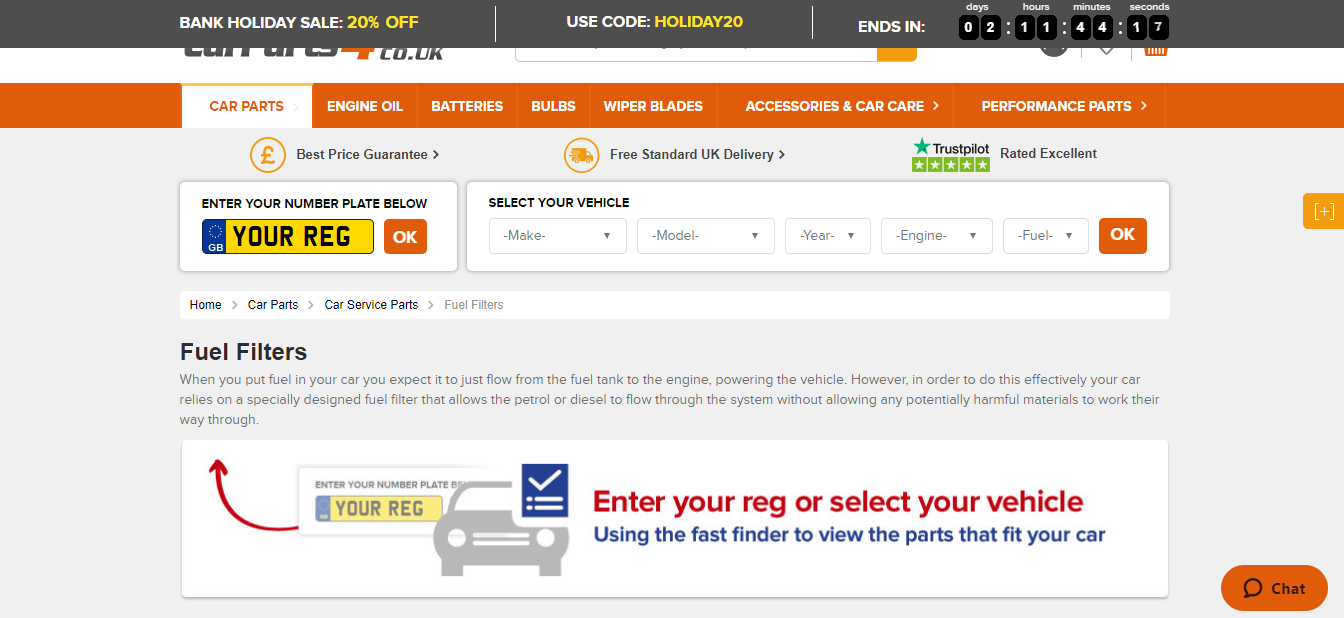**Caption:** 

The screenshot features a sleek, gray background with a prominent black-gray header. Bold white text announces a "Bank Holiday Sale" alongside a vibrant yellow "20% Off". Below, in crisp white, are details on how to redeem this offer: "Use Code: Holiday 20". The countdown timer, in white text, prominently displays the urgency with "Ends In: 2 Days, 11 Hours, 44 Minutes, 17 Seconds".

An orange header bar lists key categories in white text, each displayed over a white rectangular backdrop: "Car Parts" stands out distinctly in this section. Other categories including "Engine Oil", "Batteries", "Bulbs", "Wiper Blades", "Accessories and Car Care", and "Performance Parts", are clearly visible.

Two informative circles add value propositions: one with a Euro or Pound symbol promises a "Best Price Guarantee", and another, featuring a truck icon, advertises "Free Standard UK Delivery". 

Further enhancing credibility, the Trustpilot section with 5 green stars and "Rated Excellent" highlights customer satisfaction. A vehicle selection tool is also available, allowing users to specify "Make", "Model", "Year", and "Engine (fuel type)" to find compatible parts. Once all details are filled, an orange square button labeled "OK" completes the interaction.